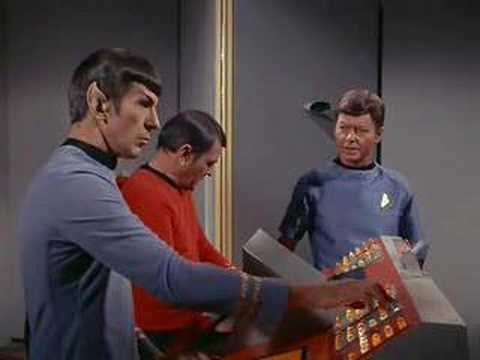In this scene from Star Trek, Spock is positioned on the left, facing toward the right. He is interacting with a machine adorned with numerous buttons. Spock is dressed in his characteristic blue-purplish long-sleeved shirt featuring a black collar. His pointed ear and neatly styled black hair are visible, emphasizing his serious expression. The background is primarily gray with a prominent yellow light extending vertically along a central door, providing a stark contrast.

In the middle, a shorter crew member with black hair and a red long-sleeved shirt, also designed with a black collar, is focused on adjusting something at the base of the machine, which necessitates his downward gaze.

To the right, another crew member, who shares the same blue-purplish uniform as Spock, stands looking concerned at his colleagues. Slightly taller than the character in the middle, this crew member has short brown hair. Numerous control panels with buttons and other intricate controls of the spaceship crafting are spread before him.

On the wall to the right, there's a small, black oblong-shaped object, possibly a button or handle, adding to the complexity of the set design.